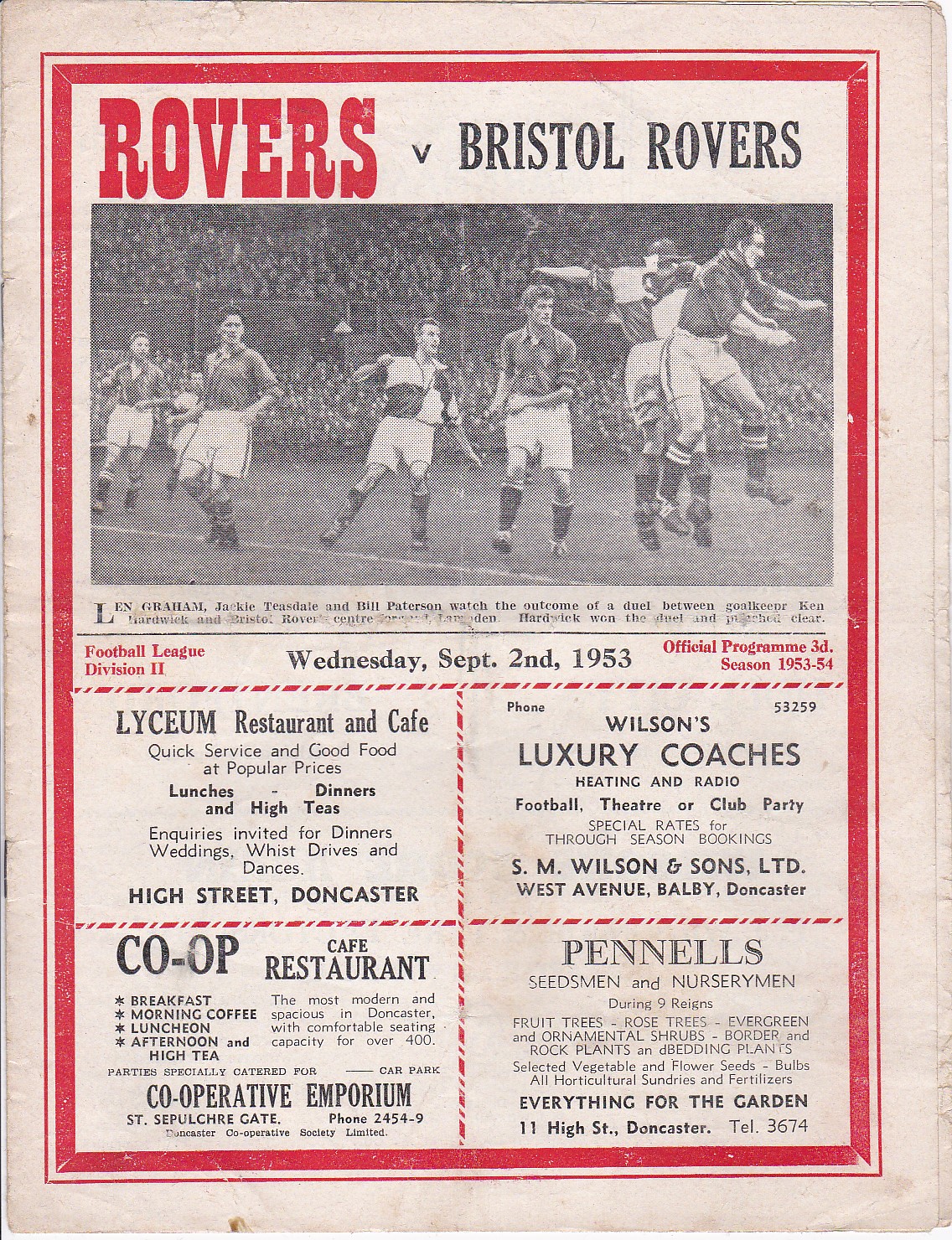This image features a historical newspaper clipping or a match program cover from September 2, 1953, advertising a soccer match between Rovers and Bristol Rovers. The worn paper is framed by a bold red border with large red lettering at the top proclaiming "Rovers" and smaller black text underneath noting "Bristol Rovers." Centrally positioned towards the top, a faded black and white photograph captures a moment of a soccer game in progress, occupying about one-third of the page. Above the image is a banner, while below it, the page is divided into four sections by a broken red line, each containing advertisements with their titles in bold black lettering. 

The advertisements include:
1. Lyceum Restaurant & Cafe
2. Wilson's Luxury Coaches
3. Co-op Cafe Restaurant and Co-operative Emporium
4. Panels for Seymour Nursery and Everything for the Garden, located at 11 High Street, with a contact number of 2614.

The background of the program is a whitish tan, and the overall content is positioned within red outlines defining the structure of the information. The style and condition of the program suggest it harkens back to a 1953 soccer match program, offering not only sporting information but also glimpses into local businesses of that era.